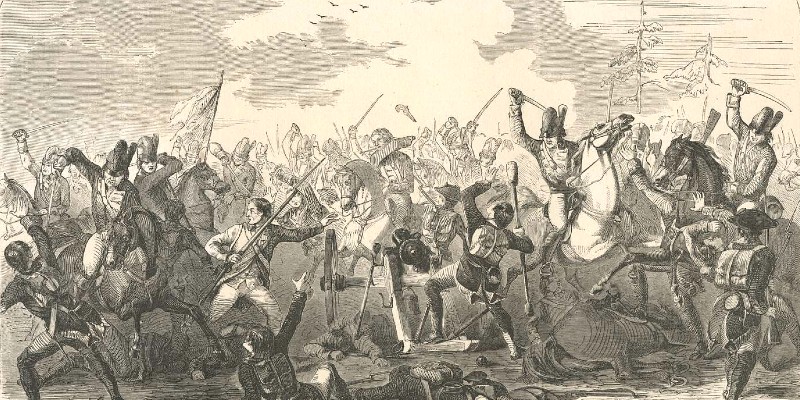A detailed pencil sketch captures a chaotic battle scene reminiscent of the Napoleonic Wars or the 1600s or 1700s. The rectangular image is horizontally oriented and primarily shaded in varying tones of gray, with the top section representing a sky filled with lightly shaded dashes, perhaps suggesting clouds or smoke. The sky also features a light tan hue and faint birds on the right, adding to the eeriness of the scene. 

In the background, there are faint images of soldiers and trees, becoming more distinct towards the middle and bottom of the illustration. Central to the scene is a dramatic interplay of combat: a man on a horse, possibly wearing a Napoleonic hat, wields a sword towards a soldier standing beside a cannon. This soldier, depicted with a round object on his neck and a large, club-like weapon, looks overwhelmed. To his left, another mounted soldier brandishes his sword, appearing ready to strike.

The battleground is densely packed with a variety of figures—soldiers on foot and horseback, some waving bayonets and flags, others wielding swords. Among them, one rider on a dark horse and another on a white horse stand out, both engaged in fierce combat. Beneath them, the ground is littered with men and horses, some lying lifeless, others in the throes of battle. A figure in a black hat stands to the bottom right, facing slightly away, adding to the sense of turmoil.

Despite the chaos, the artist has etched in hauntingly clear details, like the soldier with a backpack next to the cannon and more distant flags and trees suggesting a deeper battlefield. The overall grim scene portrays a brutal moment frozen in time, emphasizing the fierce and tumultuous nature of historical warfare.